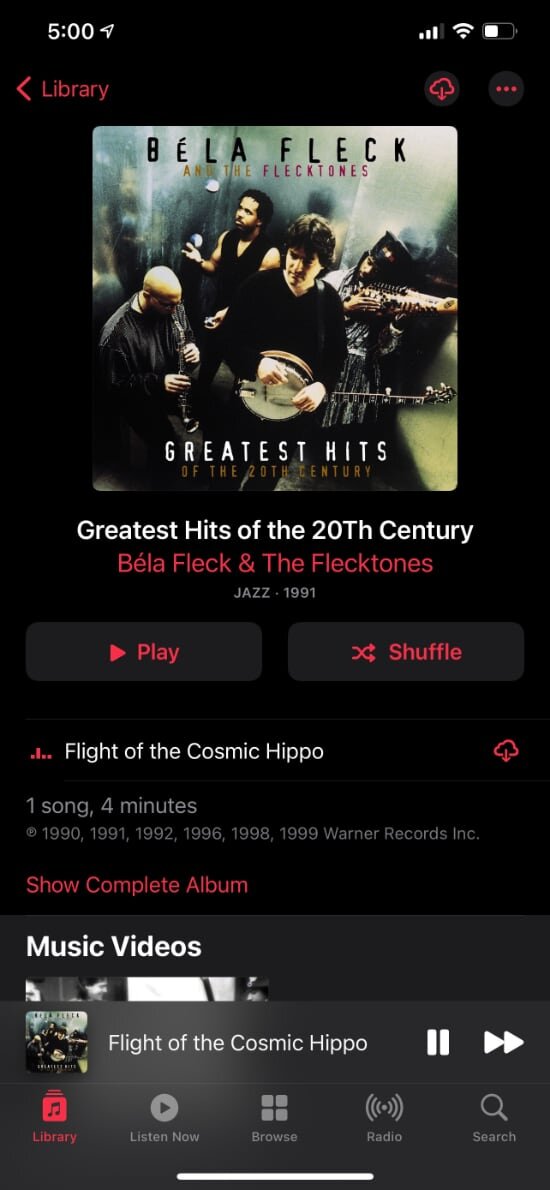The screenshot captures the interface of a music app, prominently set against a sleek black background. In the top-left corner, the time is displayed as "5:00" with a white-bordered arrow pointing diagonally upward to the right. Adjacent on the right side, the status bar indicates "3 of 4" bars for cellular signal strength, complete "3 of 3" bars for Wi-Fi connectivity, and a half-filled battery icon suggesting moderate battery life. 

Further down, the interface features a red-font navigation menu. On the left side, a left-pointing arrow is labeled "Library." Next to it, icons for downloading content and accessing more options (three vertical dots) are also highlighted in red. 

The main feature of the app screen showcases "Béla Fleck and the Flecktones - Greatest Hits of the 20th Century." An image of the band members in an elevator with mirrored walls serves as the album cover. Additional album information lists "Jazz, 1991," emphasizing the genre and release year. 

Prominent play and shuffle buttons are available for user interaction. Below these buttons, the currently highlighted song, "Flight of the Cosmic Hippo," is noted to last four minutes. Options to "Show Complete Album" and "Music Video" are provided. Playback controls for pausing or fast-forwarding are also part of the interface. 

Finally, the bottom navigation menu offers quick access to "Library," "Listen Now," "Browse," "Radio," and "Search" functions.